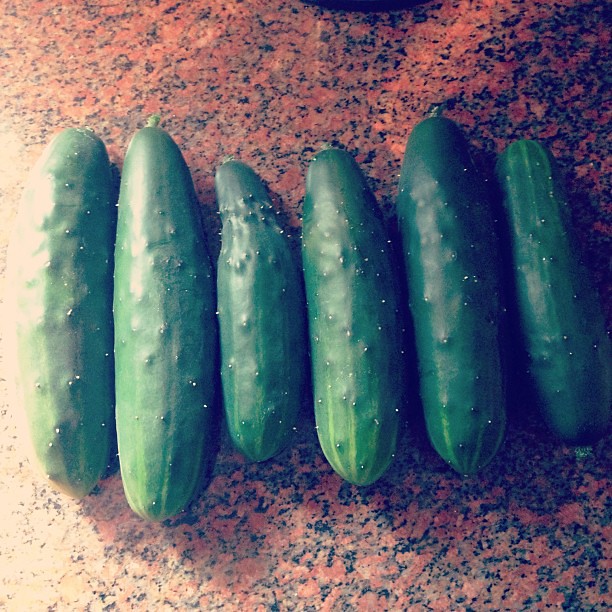This square photograph, enhanced with an Instagram filter that fades from dark blue in the upper right to tan white in the lower left, provides a top-down view of six green cucumbers arranged neatly in a row from left to right. These cucumbers, which are about six to seven inches in length, rest on a speckled, brick-red countertop made of stone or granite mixed material, featuring shades of black, gray, and a bit of white. The filter gives the cucumbers a darker than usual appearance, with their green hue transitioning from dark green at the top to a paler green at the bottom, accented by some white stripes resembling small watermelons. The cucumbers are characteristically bumpy with small raised bumps ending in white dots, and their pointed ends show slight stem remnants. The image is well-illuminated from a light source emanating from the left, casting a bright highlight on the cucumbers, emphasizing their various sizes and shapes.